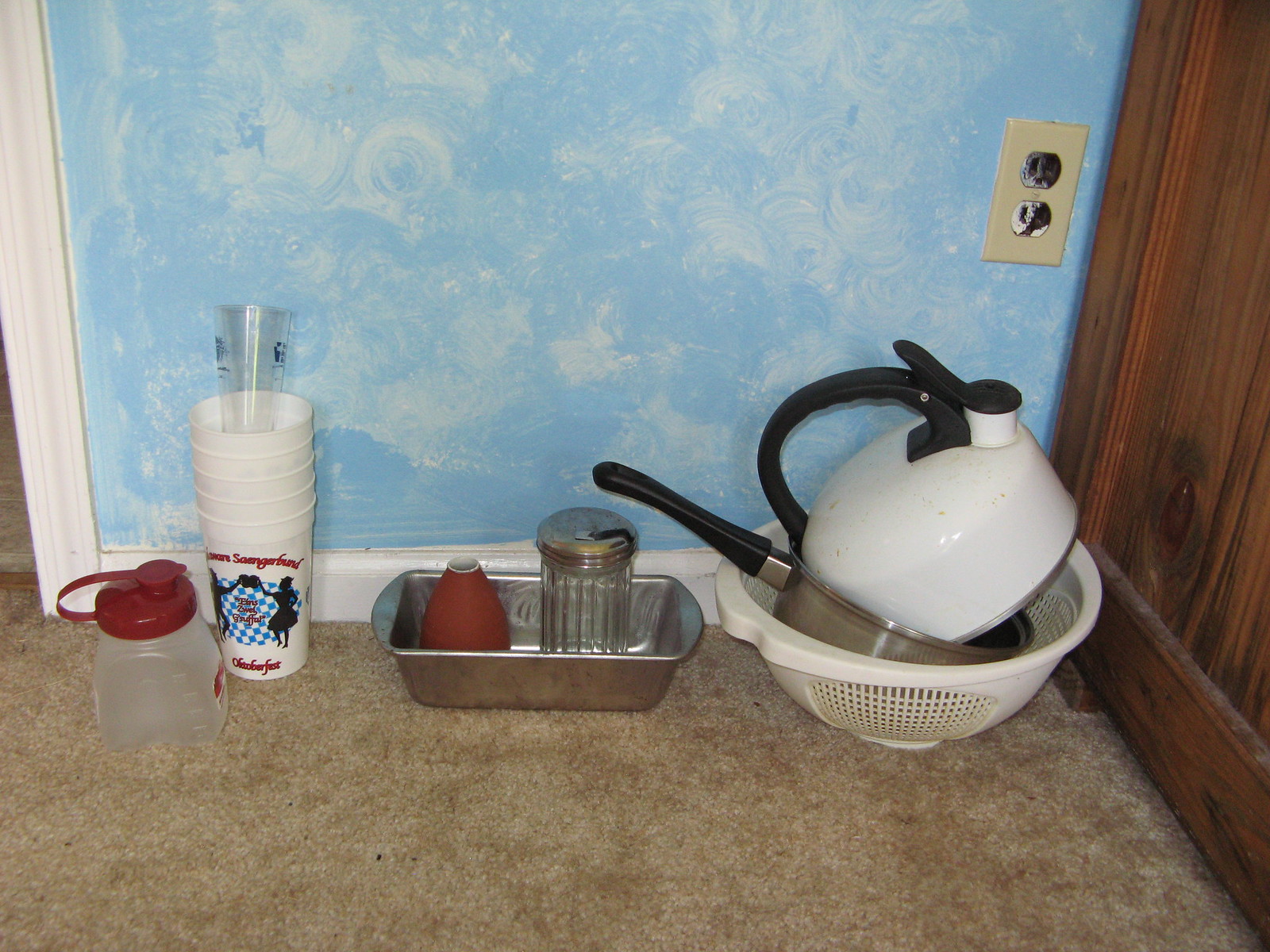The image portrays a cozy segment of a kitchen. Dominating the background is a light blue wall adorned with elegant white swirls, resembling a serene sky filled with wispy clouds. A beige electric outlet is mounted on the wall, featuring two black sockets. To the side, a brown wooden shelf is partially visible. The floor showcases a variegated pattern of light brown, dark brown, and white, complemented by white trim around the wall. A white doorway adds structure to the scene.

On the floor, a white plastic colander is prominently placed. Nearby, a silver pan with a black handle rests alongside a white tea kettle, also equipped with a black handle. A small silver loaf pan containing a red funnel-like object is part of the arrangement. A glass sugar decanter with a silver metal top and a stack of four or five white plastic cups, decorated with dancers, blue and white checks, and red writing, add to the assortment. Topping the stack is a clear plastic cup. Additionally, a small clear plastic container with a red lid is positioned among the kitchen items, contributing to the array of objects in this homey kitchen scene.